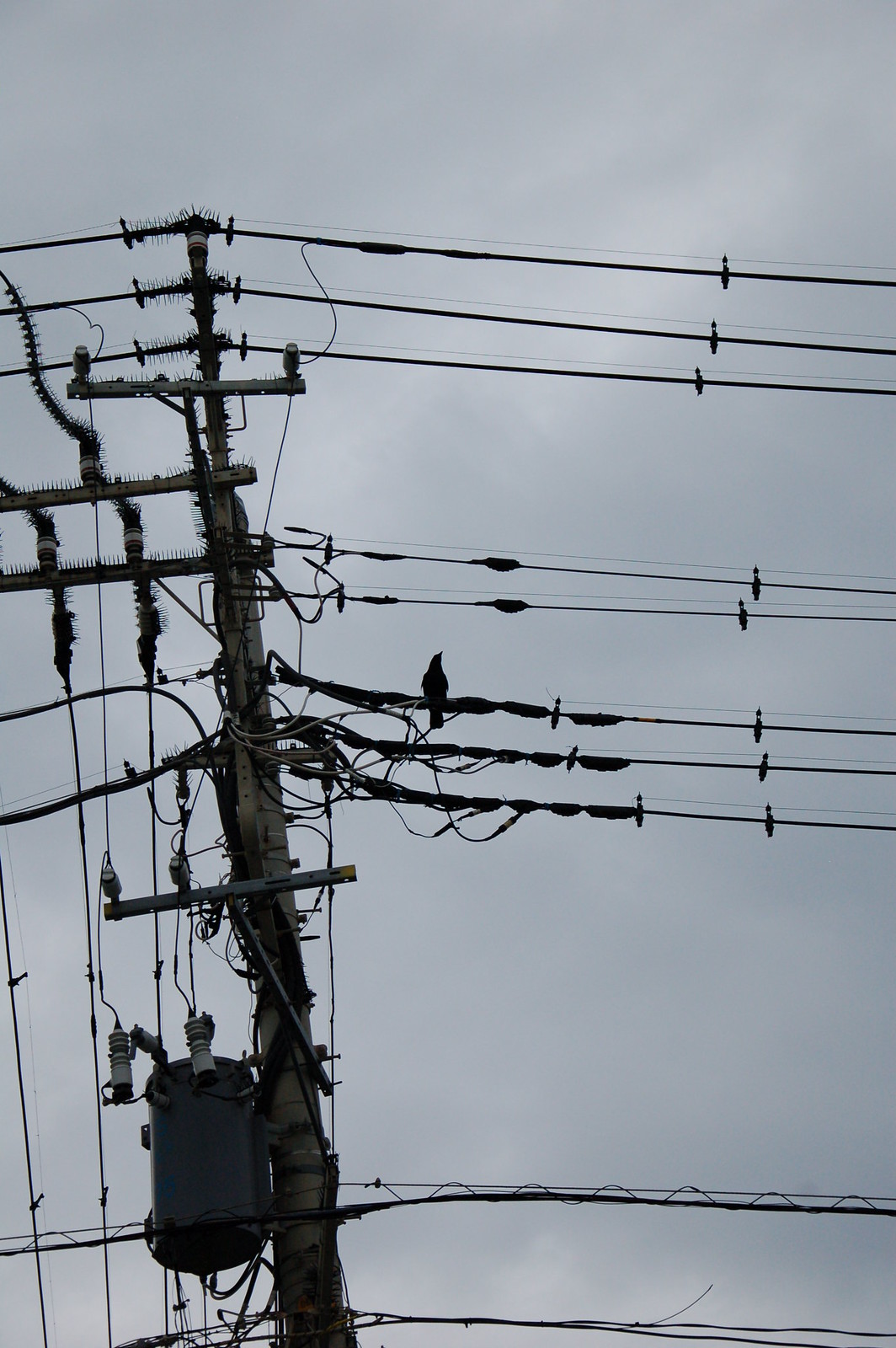The photograph captures a large wooden utility pole slightly off-center to the left, extending vertically from the bottom to the top of the frame. The sky in the background is a mix of blue-gray hues, dotted with dark clouds, lending a somber atmosphere to the scene. At the base of the pole, on the left side, there is a sizable, grayish-black electrical box. The pole is cluttered with numerous wires, creating a complex network. At the top, a trio of wires converges at the pole's center. Below them are two more wires, followed by another set of three wires, with a black crow perched on the top wire of this trio. Towards the bottom, there are two additional wires running across. Additionally, several wires run vertically on the left side of the pole. The overall composition gives an impression of a messy, interconnected web of electrical lines against a moody sky.